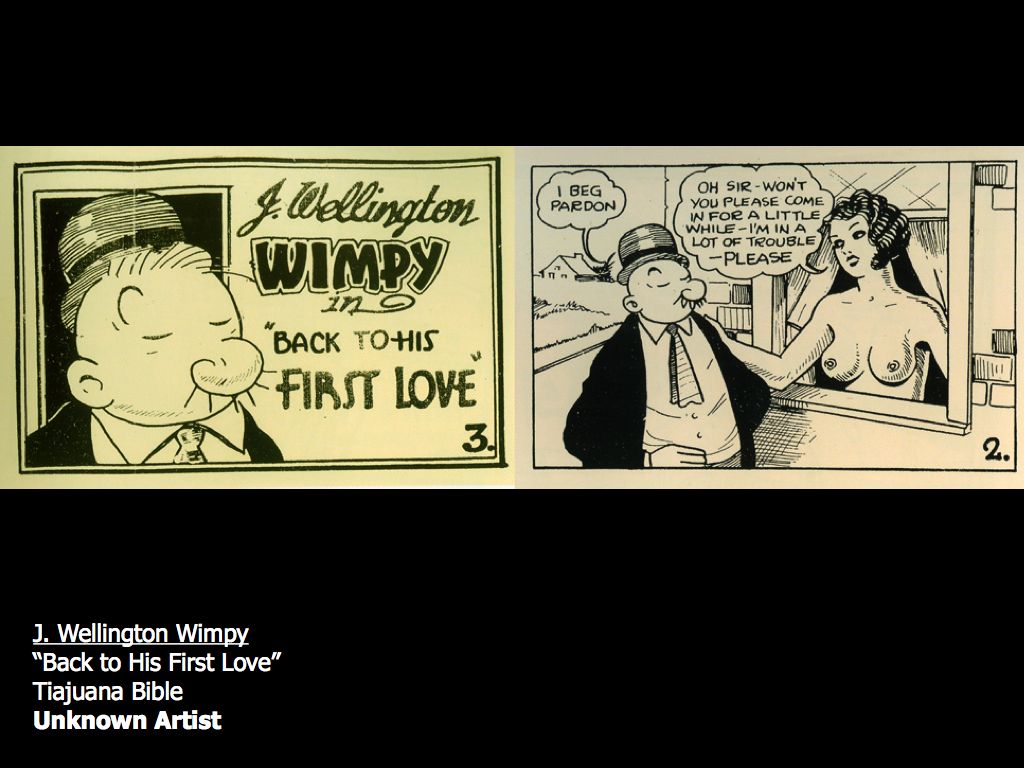A black-and-white comic strip featuring J. Wellington Wimpy from the Popeye franchise, titled "Back to His First Love." The strip is part of a Tijuana Bible, created by an unknown artist. The comic is divided into two parts. In the first panel, Wimpy, characterized by his closed eyes, large nose, and mustache, is depicted walking past a window. He is dressed in a black suit coat, tie, and white shirt. The text at the bottom of this panel reads "J. Wellington Wimpy, Back to His First Love," with the number 3 in the bottom right corner. The second panel features Wimpy encountering a nude woman leaning out of a window, her hand on his shoulder. Wimpy responds with "I beg pardon," while the woman pleads, "Oh sir, won't you please come in for a little while? I'm in a lot of trouble, please." This panel is labeled with the number 2 in the bottom right corner. The comic strip has black bars above and below the panels; the bottom bar contains the caption "J. Wellington Wimpy, 'Back to His First Love,' Tijuana Bible, Unknown Artist" in white text.